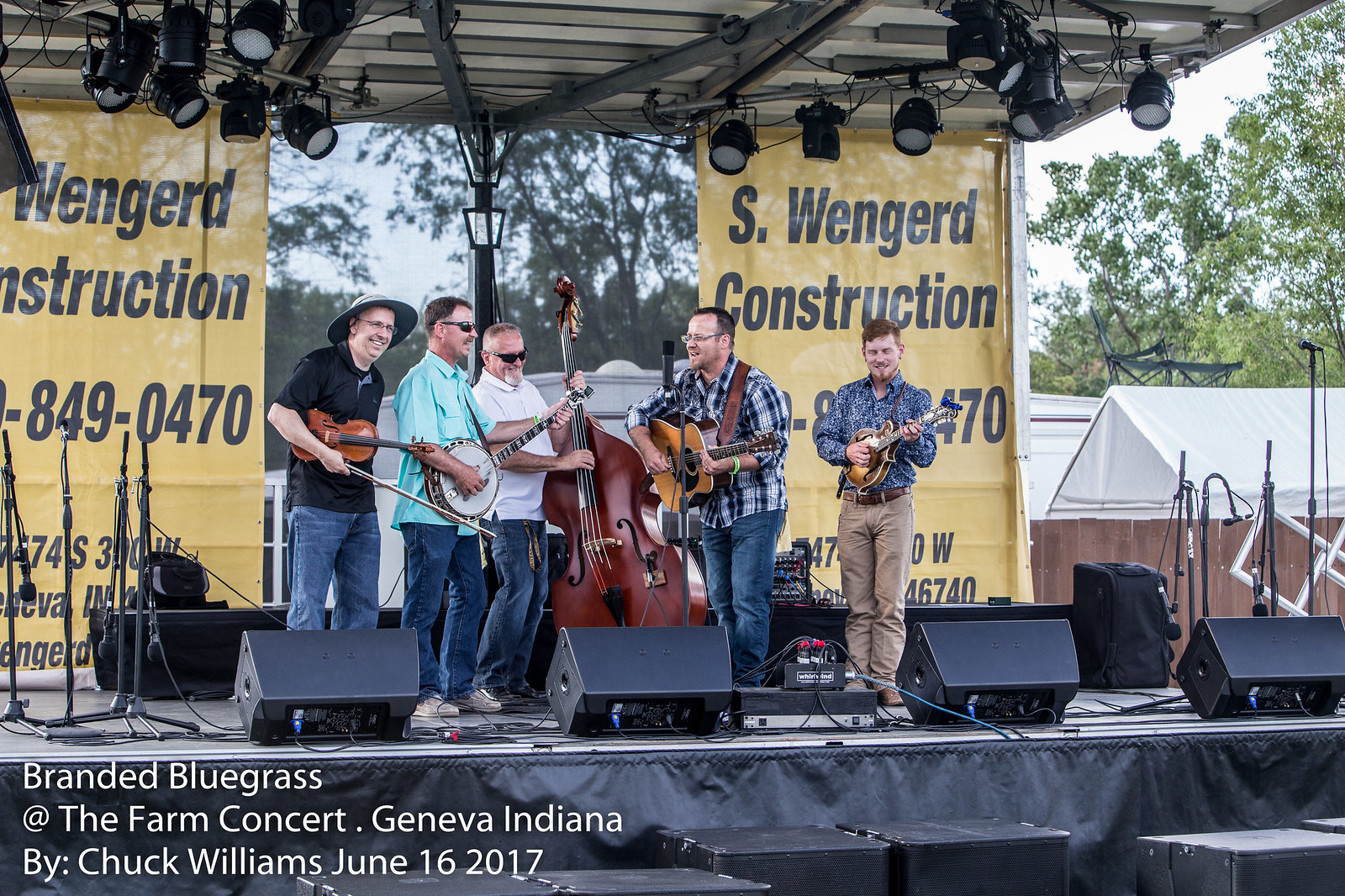The image captures a lively scene of a bluegrass band performing on stage at the "Branded Bluegrass at the Farm Concert" in Geneva, Indiana, on June 16, 2017, as noted by text in white at the bottom left corner. The stage has a black front skirt and is equipped with various stereo sound equipment and multiple mic stands. In the background, two yellow banners from S. Wingard Construction (phone number: 849-0470) flank the performers on either side. 

The band consists of five Caucasian male musicians, each immersed in their music. From left to right, we see a musician in a wild blue shirt and khaki pants energetically playing the banjo. Next to him is a man with a plaid button-up shirt and blue jeans, skillfully strumming an acoustic guitar. Center stage is a bearded man in sunglasses, wearing a white button-up shirt and blue jeans, deeply focused on playing the cello. Beside him, a musician with sunglasses, a baby blue button-up shirt, and blue jeans is deftly handling another banjo. Finally, a man in a Gilligan hat, black shirt, and blue jeans, animatedly plays the fiddle. The stage is set against a backdrop of vibrant colors, including yellow, black, and red, along with numerous spotlights hanging from the ceiling, suggesting it is a well-prepared daytime event. The entire band appears to be having a grand time, creating an infectious atmosphere of fun and music.